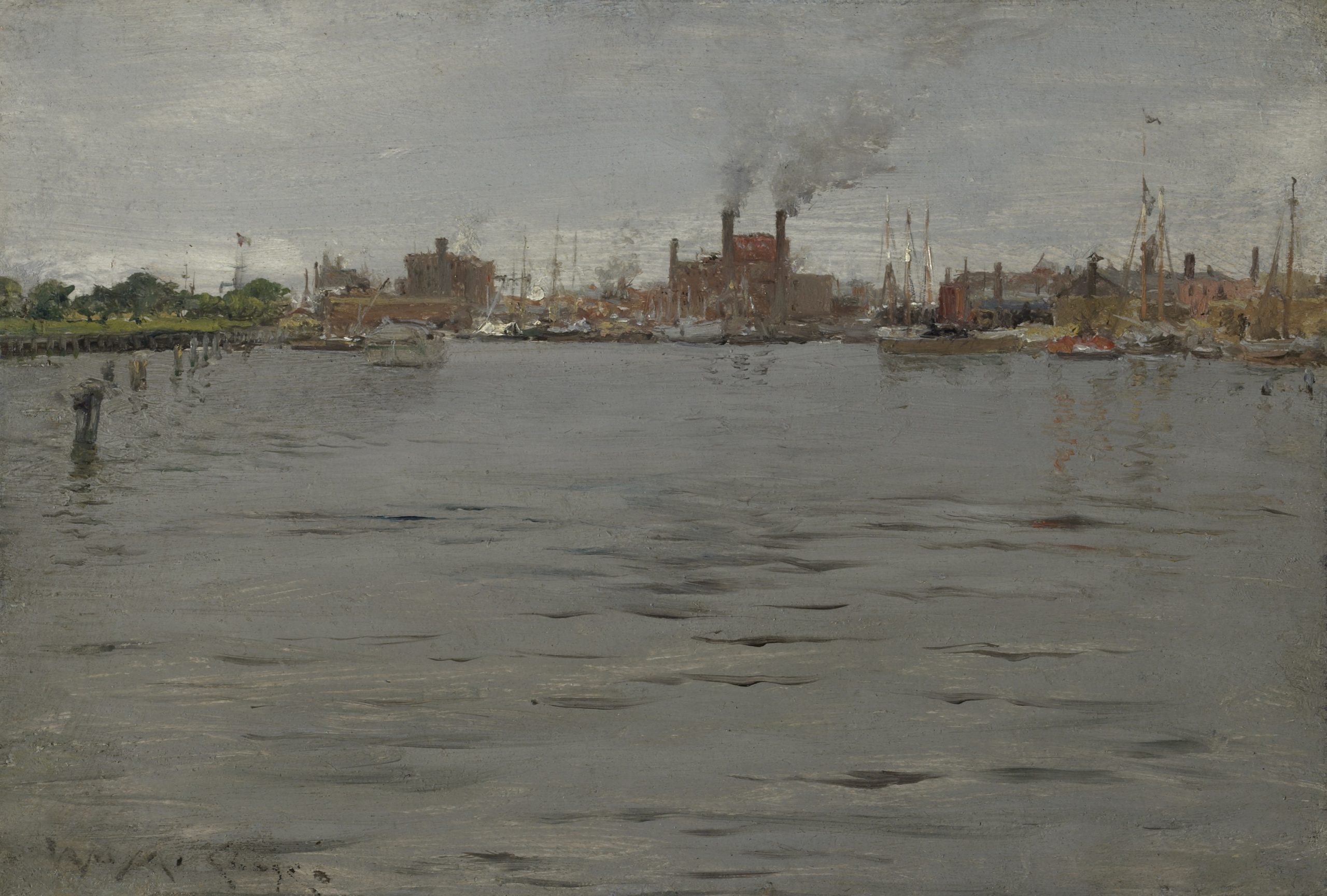The image depicts a realistic, almost painterly view of a harbor town, dominated by a gray and overcast sky. In the distance, multi-story brick buildings and factories are visible, their large smokestacks emitting whitish-gray smoke. The docks are bustling with numerous boats of various sizes, including sailboats and motorboats, with masts adorned with American flags. The harbor's water, occupying the lower two-thirds of the image, is a muted gray with small black wavelets and ripples. On the left side near the middle, some greenery, likely trees and grass, introduce the only splash of color in the otherwise monochromatic scene. Additionally, a few pillars and possibly buoys protrude from the water in this green area. The image, with a faded bluish-gray hue, also features what might be the artist's signature or inscription in the bottom left corner.